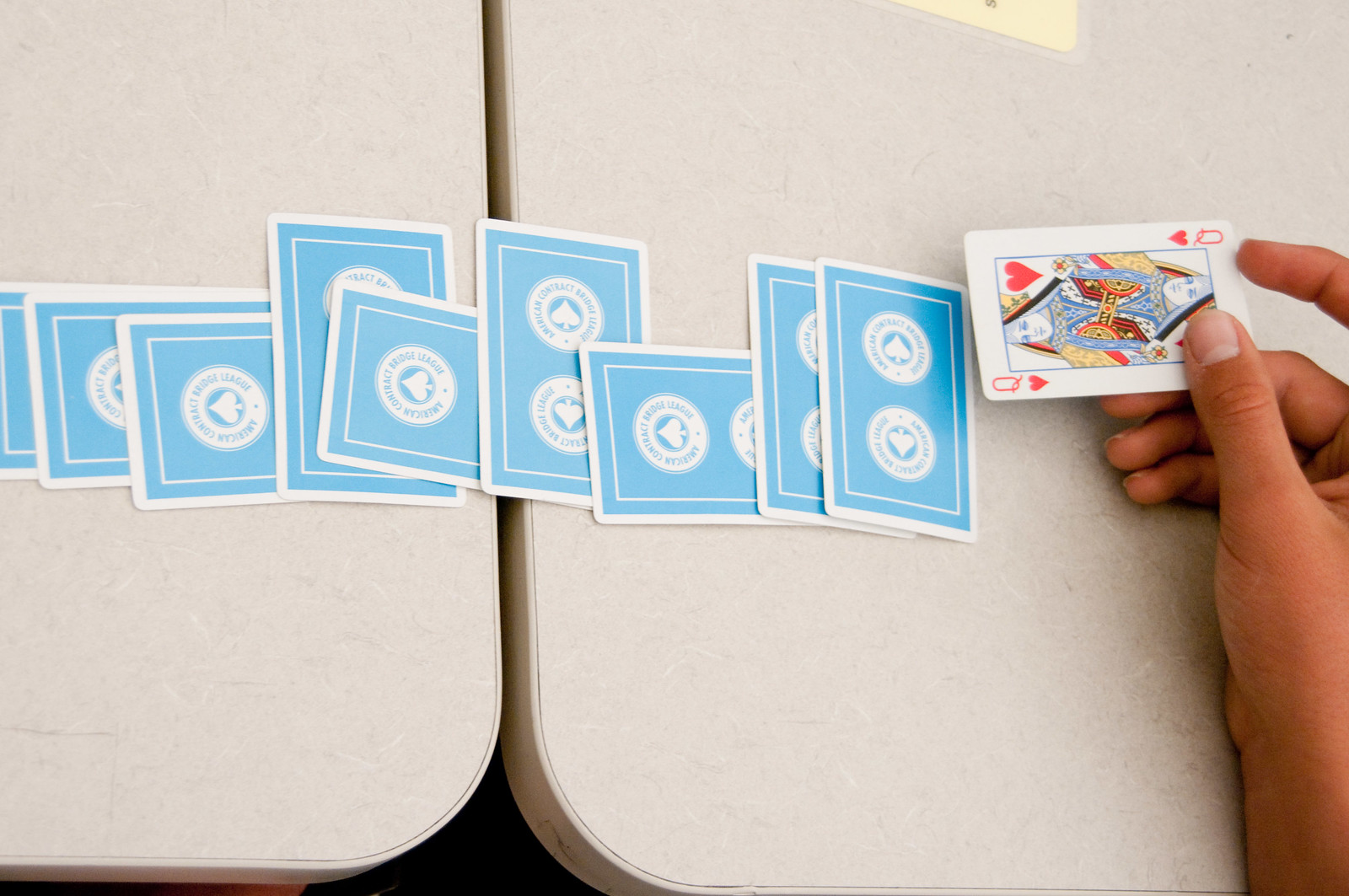In the image, we observe a meticulous arrangement of playing cards spread across two adjacent tables, which have rounded corners and a small gap of about a quarter inch between them. The focal point shows a hand in the lower right-hand corner holding a Queen of Hearts, with her face upright. Extending from this card to the left, spanning the gap and continuing offscreen, is a sequence of playing cards placed face down in a row. The card backs are light blue with a white border, featuring two round medallions, each containing a spade and some unreadable text within a white rectangle.

The cards are arranged in a specific pattern, alternating between portrait and landscape orientations. From right to left, the sequence starts with two portrait cards, followed by one landscape card, one portrait card, one landscape card, one portrait card, and finally, three landscape cards. Each card partially overlaps the next, creating a continuous, though not entirely obvious, pattern. Despite the varying orientations, the cards are aligned neatly, with none positioned diagonally.